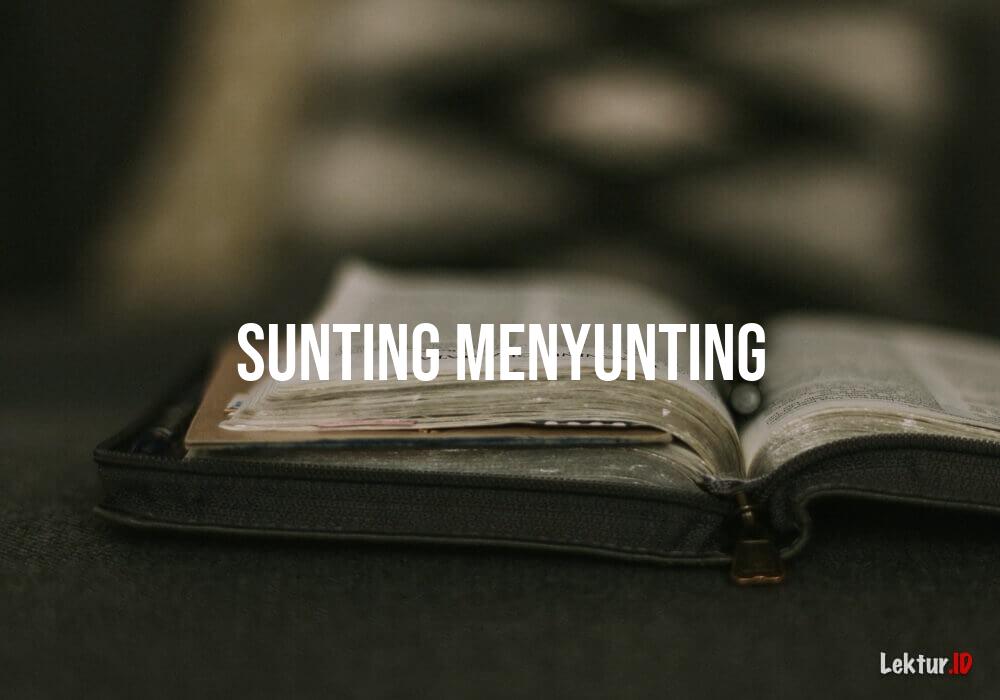The image depicts an open, weathered book, potentially a Bible, encased in a black, zippered cover with gold accents. The open book is held in place by a pen and some cardboard tabbing specific pages. The text on the pages is indistinguishable, but the edges are stained brown from age. The book is set against a dark, blurry background, possibly on a textured gray surface. Superimposed in the middle of the image are capitalized white letters that read "SUNTING MENYUNTING." In the lower right corner, "LEKTUR" is written in white, followed by ".ID" in red.